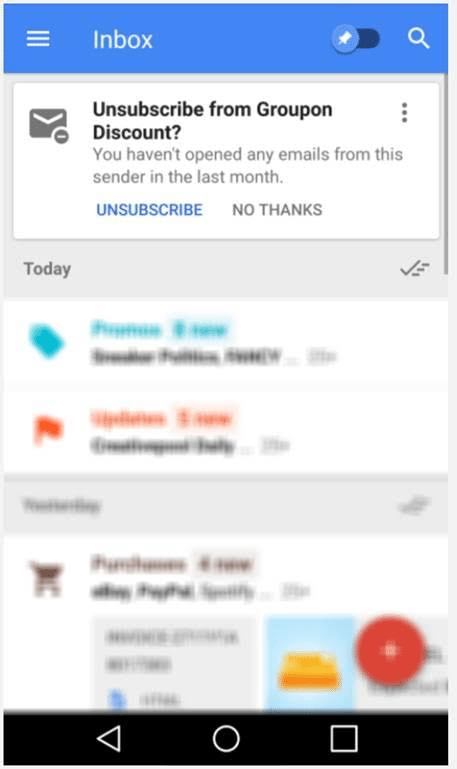The image displays a screenshot interface, most likely from an email application. At the top of the screenshot is a blue header bar with a unified blue background. On the left side of this bar is a menu icon consisting of three horizontal lines, and next to it, the word "Inbox" is displayed in white text. To the right of this is a slider bar with a circle and a pin indicating a specific position on the slider. All the way to the right end of the bar is a magnifying glass icon, indicating a search function.

Below the blue header, within a white box, is a prominent message that states "Unsubscribe from Coupon". Directly beneath this line, it reads "Discount", followed by a notification stating, "We haven't opened any emails from this sender in the last month". Below this message are two interactive options: "Unsubscribe" highlighted in blue text and "No Thanks" in dark grey text. To the left of these options is an envelope icon.

Further down, the text "Today" is displayed in a slightly greyed-out format, indicating a timestamp. Additionally, there is another box with more information, but it is also greyed out, making it difficult to ascertain the details.

At the very bottom of the image, there is a black footer bar, featuring three icons aligned to the left: a leftward-pointing triangle (likely a back button) in the center, a circle (possibly a home or main menu button) to its right, and a square with white borders. 

Overall, the screenshot appears to be from an email application, depicting a user's interaction with an email, specifically an option to unsubscribe from receiving discount coupons from a certain sender.